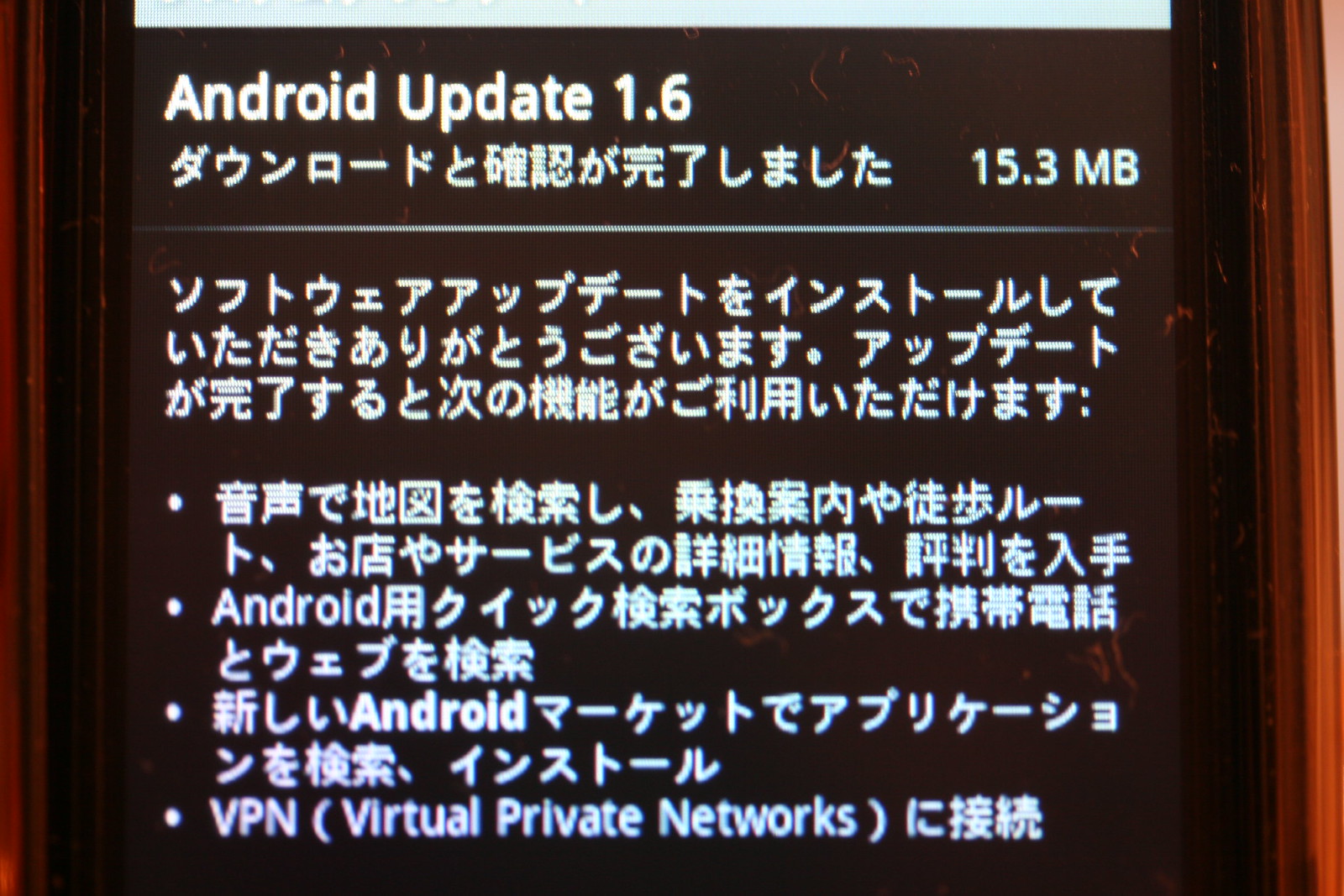The image displays the screen of an Android phone, showcasing an "Android update 1.6" notification. This text is prominently featured at the top of the screen in a bold, white font with 'A' and 'U' capitalized. The update size is specified as "15.3 MB." The majority of the text beneath the main heading is in Mandarin, including:

1. A line of Mandarin text.
2. A white line dividing the sections.
3. Three subsequent lines of Mandarin text.

Additionally, there are several bullet points listed in Mandarin. The second and third bullet points start with the word "Android" followed by more Mandarin text. The final bullet point includes "VPN (virtual private networks)" in parentheses along with some Mandarin characters. The background of the notification area appears to be brown and beveled, giving the screen an organized and framed look.